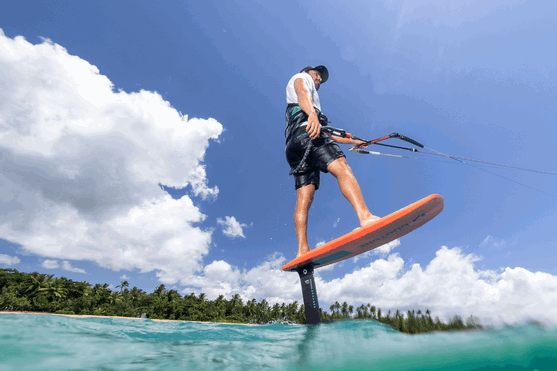In this captivating image, we see a man engaging in an exhilarating watersport activity on an electric wakeboard, which is a small, reddish-orange board elevated about a foot above the vibrant blue-green water by a black, hydrofoil-like extension. He is gripping a handled rope tethered to a boat, which is off-screen, and using only his left hand for support, while his right arm hangs down. The man, who has a beard and white skin, is dressed in black swim trunks, a white t-shirt, and a black baseball cap. The image is set against a stunning backdrop of a bright blue sky interspersed with fluffy white clouds, and the sun, though off-screen, bathes the scene in sunlight. In the distant background, a shoreline lined with trees stretches across the horizon, completing this picturesque and dynamic scene.